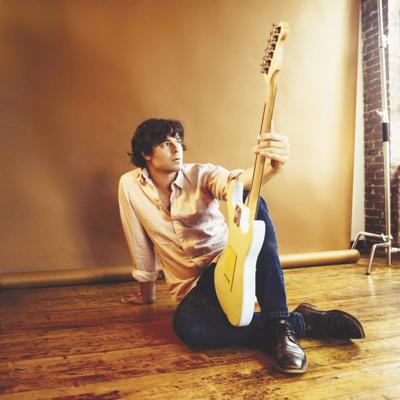The photorealistic photograph captures a man in his late 20s or early 30s, sitting on a polished hardwood floor. He has longish, curly brown hair and wears a light-colored, long-sleeved button-down shirt rolled up to his elbows, blue jeans, and brown reflective dress shoes. With a naturalistic lighting setup illuminating the scene more brightly on the right side, he sits in front of a light tan unfurlable backdrop, partially revealing a section of exposed brick wall. His seating position is casual; his left leg is raised and bent at the knee, while his right leg is crossed and resting on the floor. He leans back on his right hand for support, his palm flat against the floor, and holds a white guitar by its neck in his left hand, positioned between his legs with the guitar's body leaning against his left leg. To the right, there is a glimpse of a photography light stand and a hint of a window, adding an authentic feel to the image.